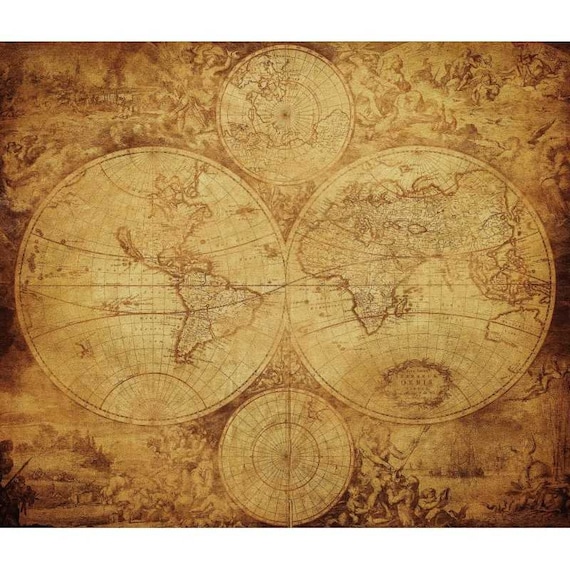The image depicts an elaborate, antique world map characterized by a sepia-toned, weathered aesthetic. Four main globes feature prominently: two large ones in the center representing the Western and Eastern Hemispheres, with North and South America on the left, and Africa, Asia, Australia, and Antarctica on the right. A smaller globe at the top presents a view from the North Pole, while an equally sized globe at the bottom displays a view from the South Pole. The margins of the map are adorned with intricate, sepia-toned artwork, including detailed silhouettes of people and mythological creatures, some with wings, depicted in various, often warlike, situations. The map incorporates decorative accents, labeled latitude and longitude lines, and the prime meridian. Also, there is some illegible writing at the bottom, contributing to its sense of historical depth and authenticity.